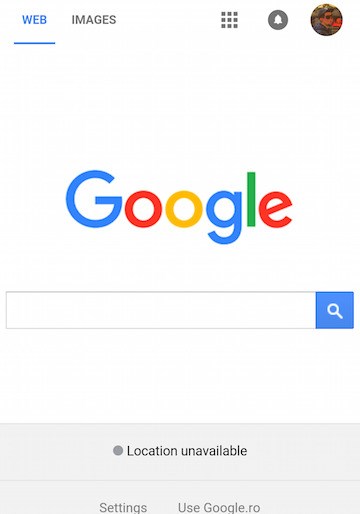The image features a detailed layout of a web interface. In the top left corner, the word "WEBB" is prominently displayed in blue, all caps, and underlined in blue. Adjacent to this, the word "IMAGES" appears in gray, also in all caps. 

To the right of these words, there is a 3x3 grid of equally spaced squares, collectively forming a larger square. Below the grid, a gray circle houses a white bell icon, symbolizing notifications. Next to it, there's a circular icon representing a user profile, indicated by a man’s silhouette.

Dominating the central area is the iconic "Google" logo. The "G" is in blue, followed by two lowercase "o"s in red and yellow, respectively. The "g" matches the blue of the initial "G," while the "l" is green, and the "e" is red, completing the familiar color scheme.

Beneath the logo lies a gray-outlined rectangular search box with a white interior. At the box's far right end, there is a smaller blue square featuring a white magnifying glass, denoting the search function.

Further down, two horizontally-aligned rectangles are separated by a thin gray line. The upper rectangle contains the text "Location Unavailable" accompanied by a gray dot to its left. Below this, the lower rectangle holds the text "Settings," followed by a space, and then "Use Google.ro," suggesting the regional version of Google's settings.